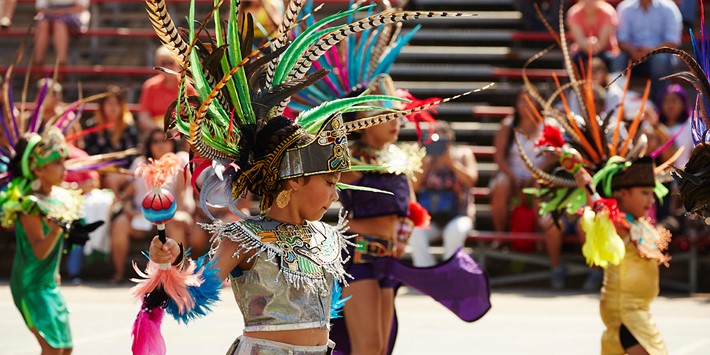The photograph captures a vibrant outdoor cultural performance featuring several young women of likely Indian descent, all adorned in intricate and colorful tribal outfits. The central figure, slightly left of center in the frame, stands out in a dazzling silver crop top paired with a matching skirt. She holds a red and blue maraca with pink flowers emerging from its top, and her wrists are decorated with blue and pink feathered bands. Her ornate headdress is a striking combination of green, brown, and long white feathers with brown stripes. Surrounding her are other young women, similarly arrayed in traditional attire that includes headdresses with a spectrum of feathers—ranging from bright oranges, purples, and blues to green feathers with black stripes. Each performer faces to the right, dancing in unison, while a blurred background reveals metal bleachers filled with onlookers, emphasizing the grand scale and celebratory atmosphere of the event.